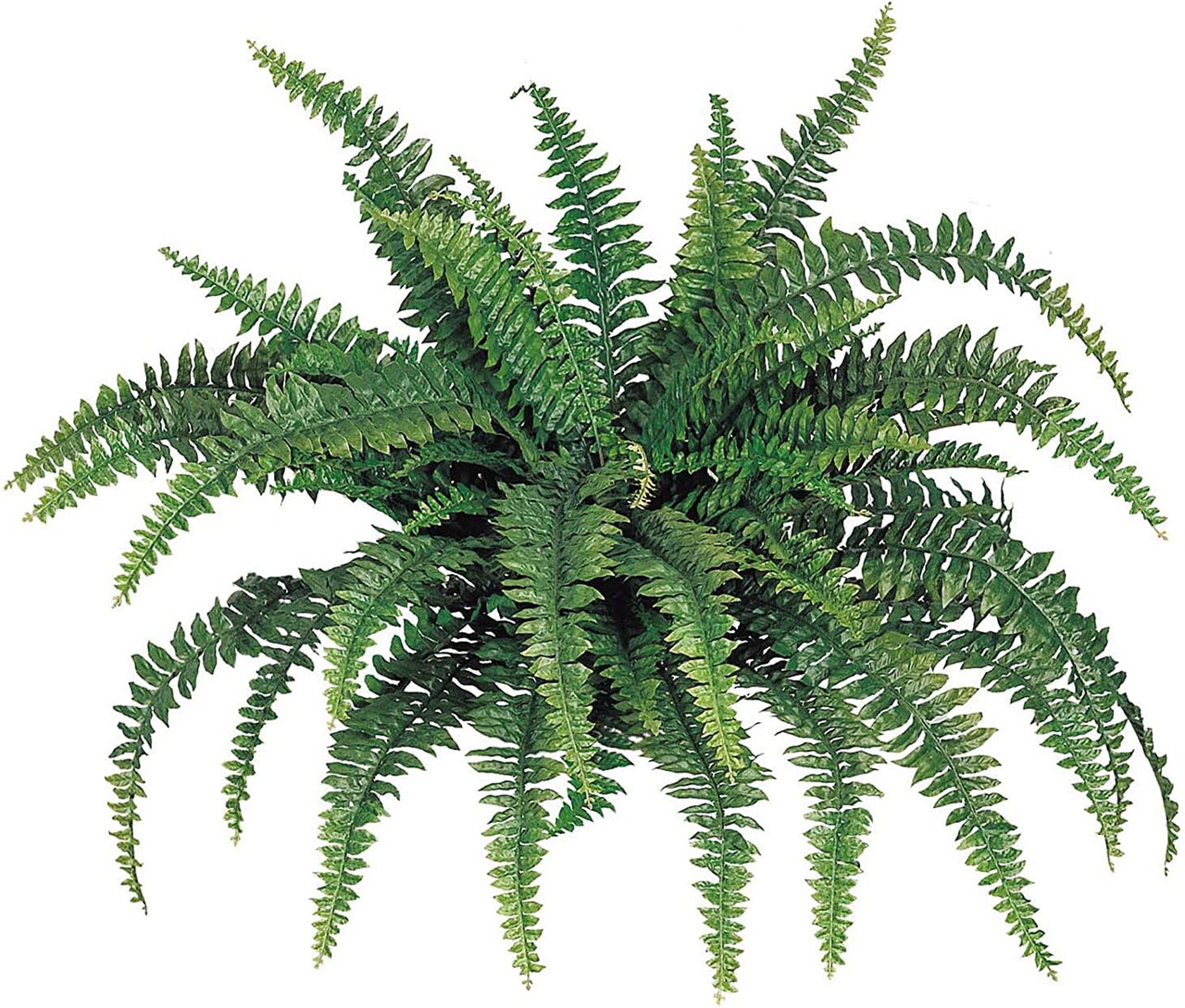The image is a photorealistic depiction of a house fern, centered against a pure white background, giving it a floating appearance. Dominating approximately 80% of the composition, the fern presents a lush display of over 40 thick fronds radiating in all directions—up, down, and to the sides. The vibrant plant showcases a spectrum of greens, with some fronds transitioning to lighter yellows and browns toward their tips, indicating age or variable watering. Despite its mature appearance, the fern looks healthy, with no visible parasites or signs of distress, exuding a naturalistic charm under soft, realistic lighting.